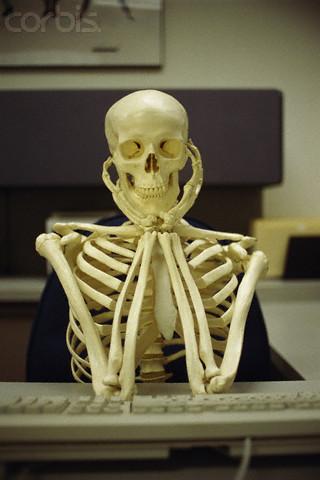This image features a skeleton posed humorously at a keyboard, evoking a sense of timeless waiting. Starting from the bottom, a thin strip of a wooden table, approximately half an inch, is visible. Situated above it is a slightly out-of-focus keyboard with an eggshell white hue, displaying its top rim and a portion of the keys. A cord emerges from the right side of the keyboard, about two inches from the edge, trailing off the image.

The skeleton, facing directly towards the camera, is seated in a blue chair. Its anatomy is fully visible, including prominently detailed ribs, arms, skull, eye sockets, and nose, with an intact set of teeth. The skeleton's arms are positioned such that it props its chin on its bony hands, giving an impression of contemplative patience.

On the image's right side, a patch of white floor is visible, while on the left, a section of a brown desk can be seen. The background, though slightly out of focus, reveals more details: a brown wall or possibly another desk extends upwards, meeting a tan wall in the top left corner. A poster inscribed with the word "Corbis" is adhered to the tan wall. Additionally, a stretch of tan flooring and a white wall occupy about a quarter of the image at the bottom. Above the skeleton's right shoulder rests a manila envelope in a black basket, adding another layer of mundane office detail to this quirky scene.